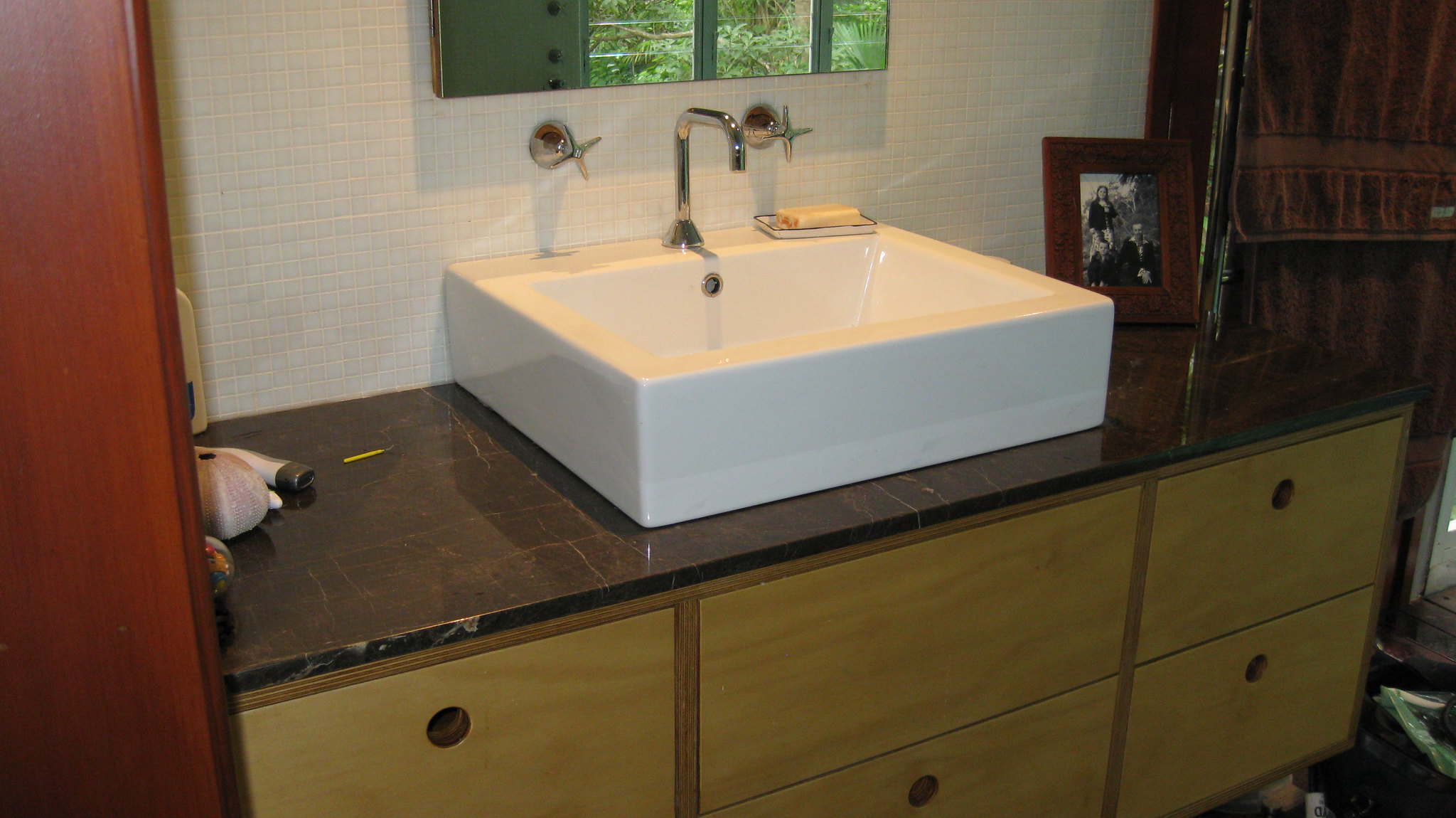This image showcases a rustic, yet charming bathroom setting highlighted by a large, square, white farmhouse sink. The sink, crafted in a strikingly pristine white porcelain, is paired with a sleek silver faucet featuring dual wall-mounted handles. The faucet's shining metallic finish provides a contemporary contrast to the classic farmhouse aesthetic. The sink is distinctly elevated, resting atop an antique, bleached or light maple wood dresser which has been repurposed as a vanity. This dresser lacks traditional knobs, opting instead for simple, functional holes to open the drawers.

The countertop of this dresser appears slightly blemished at the lower left corner. The backdrop features a classic tiled backsplash enhancing the rustic appeal of the space. On the right side of the backsplash, there is a small, framed picture, adding a personal touch to the room. Meanwhile, on the left, a mysterious tube is present, whose purpose is not immediately clear.

To the extreme right of the image, a towel is visible, suggesting this is indeed a bathroom rather than a kitchen. Furthermore, the presence of a potential mirror on the right side implies a space dedicated to personal grooming. The overall ambiance of the space combines rustic elements with functional modern details, creating a warm and inviting bathroom setting.